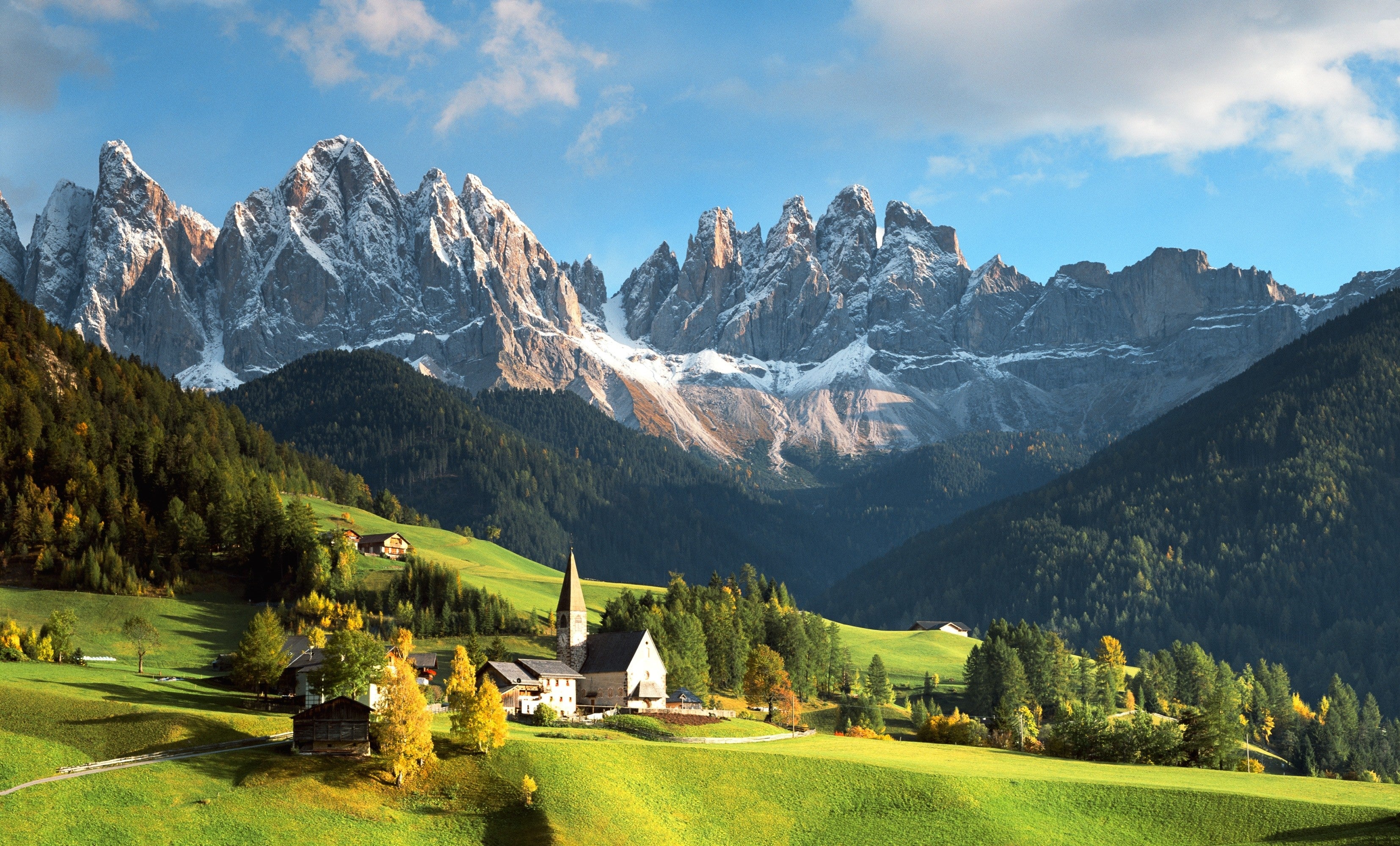In this picturesque countryside image, we see a breathtaking spring day with a light blue sky adorned with drifting white and gray clouds. The background is dominated by majestic, snow-capped mountains, showcasing a blend of gray and brown rocky terrain with patches of white snow. Rolling green hills extend towards the foreground, creating a vibrant and inviting landscape. The lush green grass at the very front is complemented by various types of shrubbery and trees, including a couple of yellow trees on the left-hand side. Prominently featured in the center-bottom of the image is a quaint, older-style white building with a black roof and a tall, pointed white steeple, which suggests it may be a church. This structure is framed by additional small buildings and a meandering road that traverses the hillside. The overall scenery evokes a serene and timeless beauty, capturing the harmonious coexistence of man-made and natural elements.